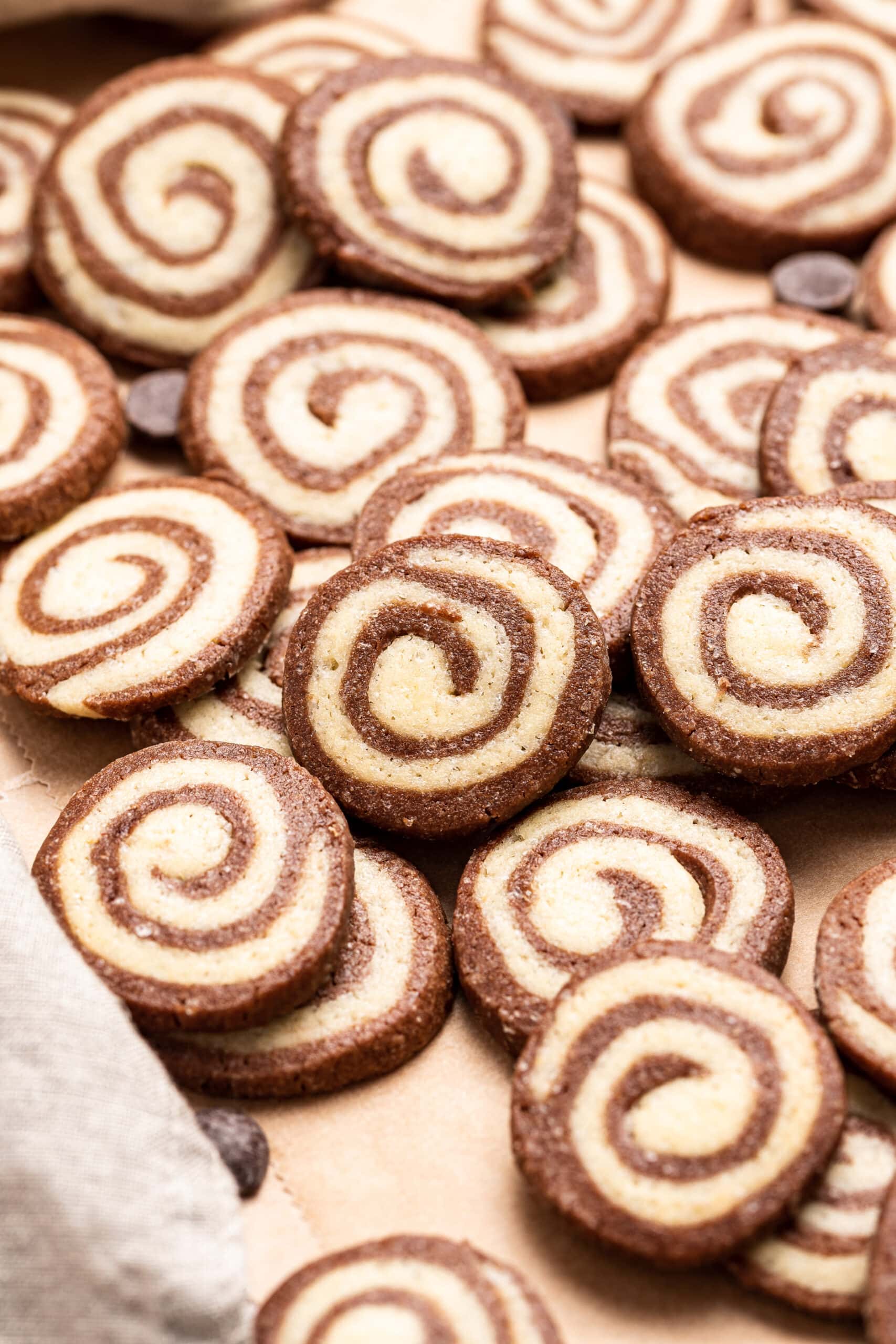This close-up image depicts a tray densely populated with approximately 20 to 30 circular cookies, uniformly baked with a distinctive spiral pattern. The cookies have a dark brown outer ring that swirls inward, transitioning into a lighter tan color at the center. The surface of each cookie is adorned with small white sugar crystals, giving them a slightly glittering appearance. The cookies are laid out on what seems to be a piece of brown parchment paper, which serves as a baking sheet. Interspersed among the cookies, there are a few small, dark brown circles resembling chocolate chips or mini Hershey Kisses, but none of these chocolate pieces are actually on the cookies themselves. Additionally, at the bottom left of the image, a piece of off-white or gray cloth is visible, adding a touch of texture to the scene.